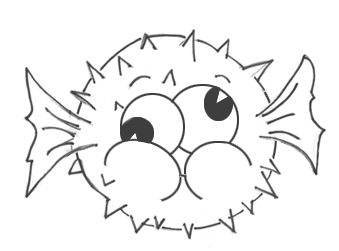This simple yet charming line drawing depicts a cartoon puffer fish on a white background. The puffer fish is essentially a round circle bristling with spikes, which even extend above its large, expressive eyes. These eyes, distinguished by contrasting black pupils, add a whimsical touch as they gaze in opposite directions—one looking up to the upper right and the other down to the lower left. Above the eyes are two curved lines that serve as playful eyebrows.

The fish's face features pronounced, semicircular cheeks at the bottom, giving the impression that it's puffing up, as puffer fish do. Adding to its quirky appearance, it has two side fins, humorously resembling bat wings, protruding symmetrically from the middle of its body. Overall, the art beautifully captures the cartoonish essence and exaggerated features typical of a puffer fish, making it appear both puffy and endearing.